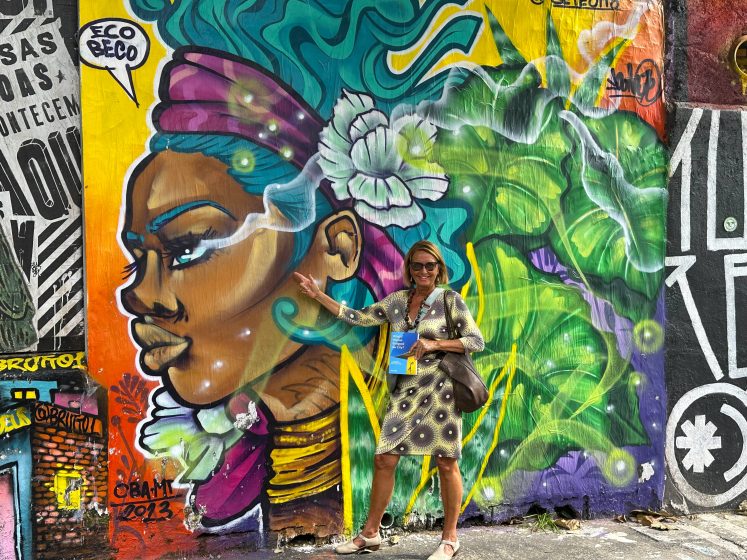In this vibrant scene, a middle-aged Caucasian woman, likely around 40 and sporting a fashionable yellow and brown wrap dress with a circular pattern, stands central to the frame. Her short, dark blonde bob frames her face adorned with dark sunglasses and subtle earrings, while a brown handbag rests over her shoulder. She wears flat sandals on her tanned, bare legs and holds a small book or travel brochure in one hand. Her other hand is outstretched, pointing at an exquisite mural behind her.

The mural itself, a stunning piece of wall art, features a striking black woman with blue eyebrows and teal-colored hair adorned with a purple headband. Her lips are pursed as smoke-like tendrils emanate from her eyes, creating an otherworldly aura. The background bursts with a medley of vivid green 3D flowers and stars, adding depth and richness to the scene. In the lower left corner, the artist's signature and the year 2023 can be discerned. Completing the mural is a speech bubble near the woman's head, bearing the phrase "Echo Beko." The woman's presence and the mural's dynamic design create a captivating contrast and a tale of discovery and travel.